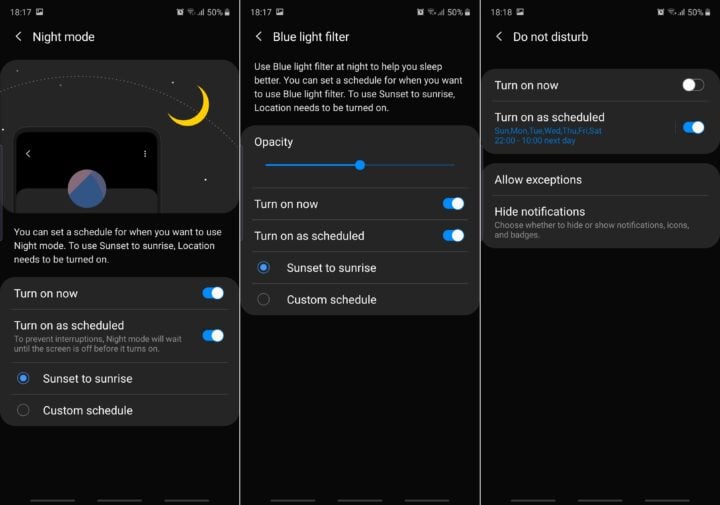The image consists of three smartphone screenshots displayed side by side, each depicting different settings for managing evening and night features.

**Screenshot 1 (Left):**
- **Time:** 18:17
- **Battery:** 50% (upper right)
- **Top Header:** Night Mode
  - A gray rectangle at the top features a yellow quarter moon icon in the upper right and what appears to be a depiction of Earth at the bottom.
  - Below it states the ability to set a schedule for Night Mode.
  - A message indicates that to use "Sunset to Sunrise," location services must be turned on.
  - Two toggle options: "Turn on now" and "Turn on a schedule" – both are enabled.
  - The selected schedule option is set to "Sunset to Sunrise."

**Screenshot 2 (Center):**
- **Time:** 18:17
- **Battery:** 50% (upper right)
- **Top Header:** Blue Light Filter
  - It suggests enabling the Blue Light Filter at night to improve sleep.
  - Similar to the first screenshot, users can set a schedule for this feature.
  - Again, using "Sunset to Sunrise" requires location services.
  - Below, an adjustable opacity slider is present, set to the middle.
  - Two toggles: "Turn on now" and "Turn on a schedule" – both are enabled.
  - The chosen schedule option is "Sunset to Sunrise."

**Screenshot 3 (Right):**
- **Top Header:** Do Not Disturb
  - The "Turn on now" toggle is disabled.
  - The "Turn on a schedule" toggle is enabled.
  - Below these options are "Allow exceptions" and "Hide notifications."

This detailed setup optimizes the phone's display and notification settings for evening and nighttime use, enhancing user comfort and ensuring better sleep by reducing exposure to disruptive lights and notifications.